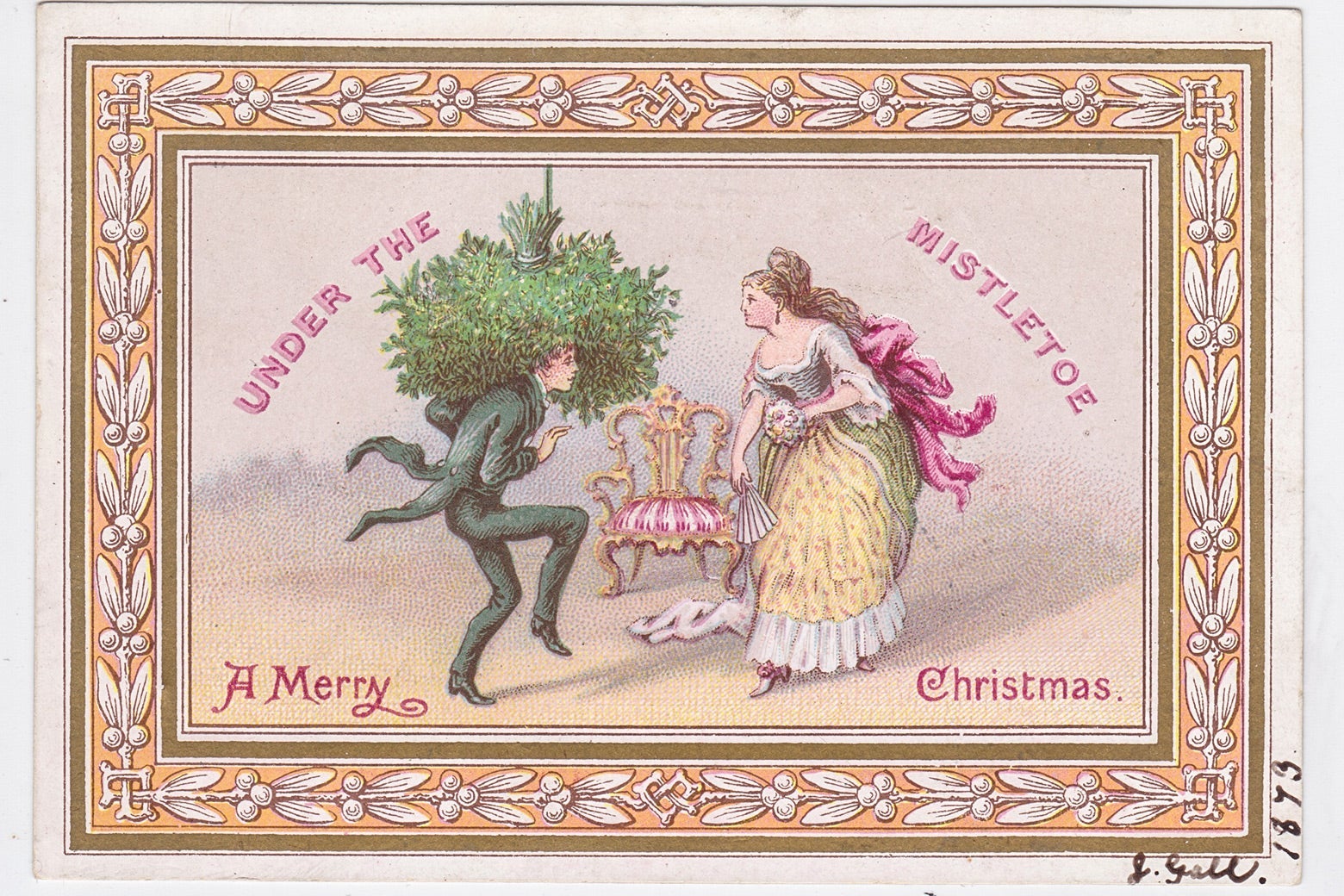This detailed painting, dated 1873 as inscribed in black on the bottom right corner, is encased in an elaborate, gold and peach-colored painted frame adorned with leaves and white berries, cleverly incorporated as an intrinsic part of the artwork. Central to the piece, a well-dressed couple takes the viewer back to the 1700s. The man, positioned on the left, is dressed in a black suit with coattails and a large bush of mistletoe atop his head. His right leg is comically raised. To his right, a woman with long brown hair, adorned with a pink ribbon, stands poised in a striking dress. The dress features white sleeves, green sides, and a yellow bottom with red dots, complemented by a red cape. She holds a white fan in her right hand and a bouquet in the same hand. Between them is an ornate gilt chair with red and white upholstery. Scattered text around the couple reads "Under the Mistletoe" in pink at the top, and "A Merry Christmas" in red text, positioned at the upper left, lower left, and lower right respectively, creating an enchanting holiday scene.